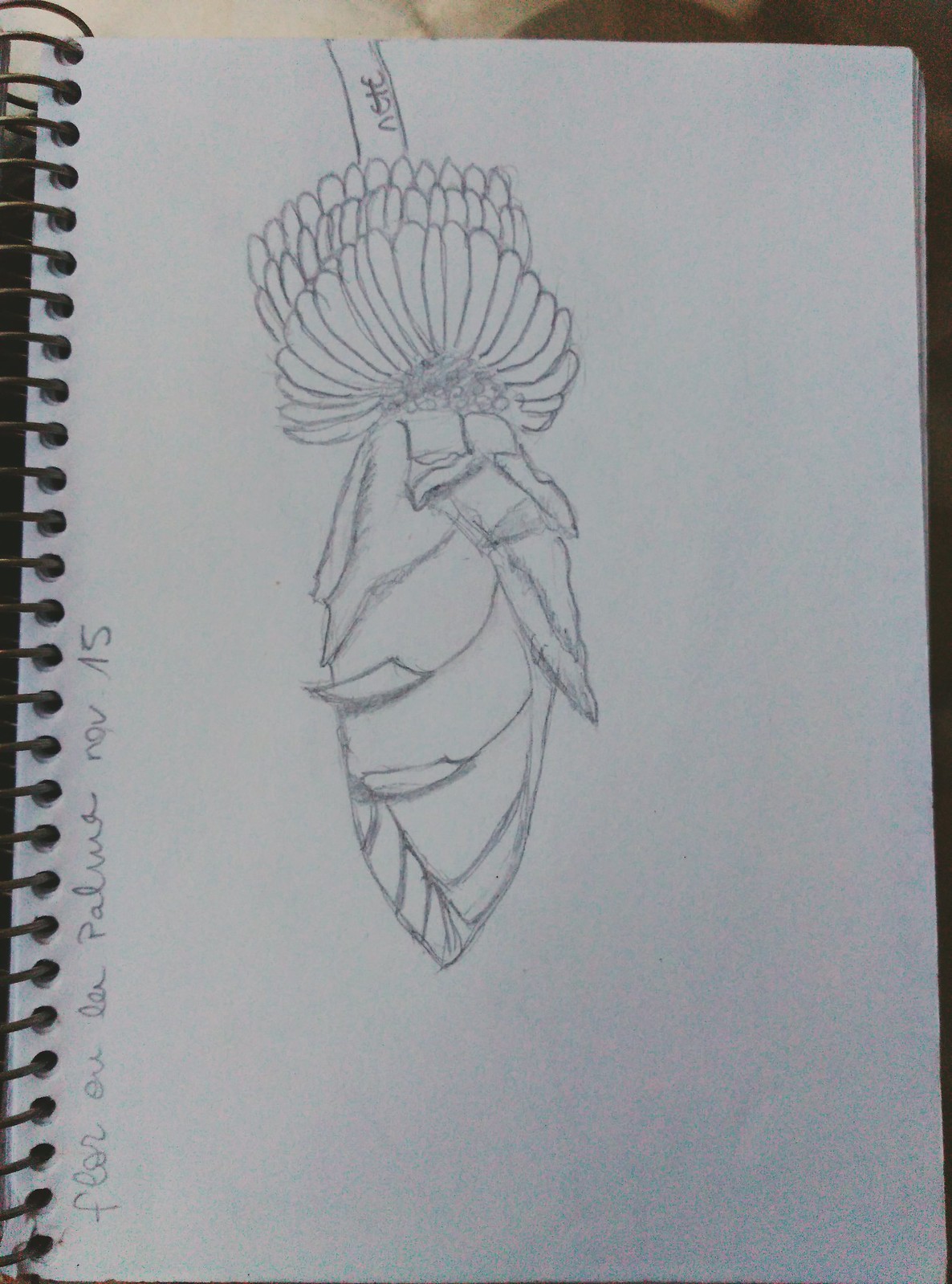In the photograph, a sketchpad lies open with its left side tucked beneath the right. Bound by a spiral on the left, the sketchpad's pages are held securely together. The focal point of the image is a detailed pencil drawing displayed on the top page. The drawing features a cluster resembling a pod of bananas arranged in three distinct rows. From this cluster, an intricate structure extends downward, tapering to a point and composed of different layered elements that add complexity to the illustration. Along the spine of the notebook, text is partially visible, reading "November 15th," preceded by four words that are difficult to decipher. The overall composition of the photograph highlights both the artistic sketch and the physical attributes of the sketchpad itself.